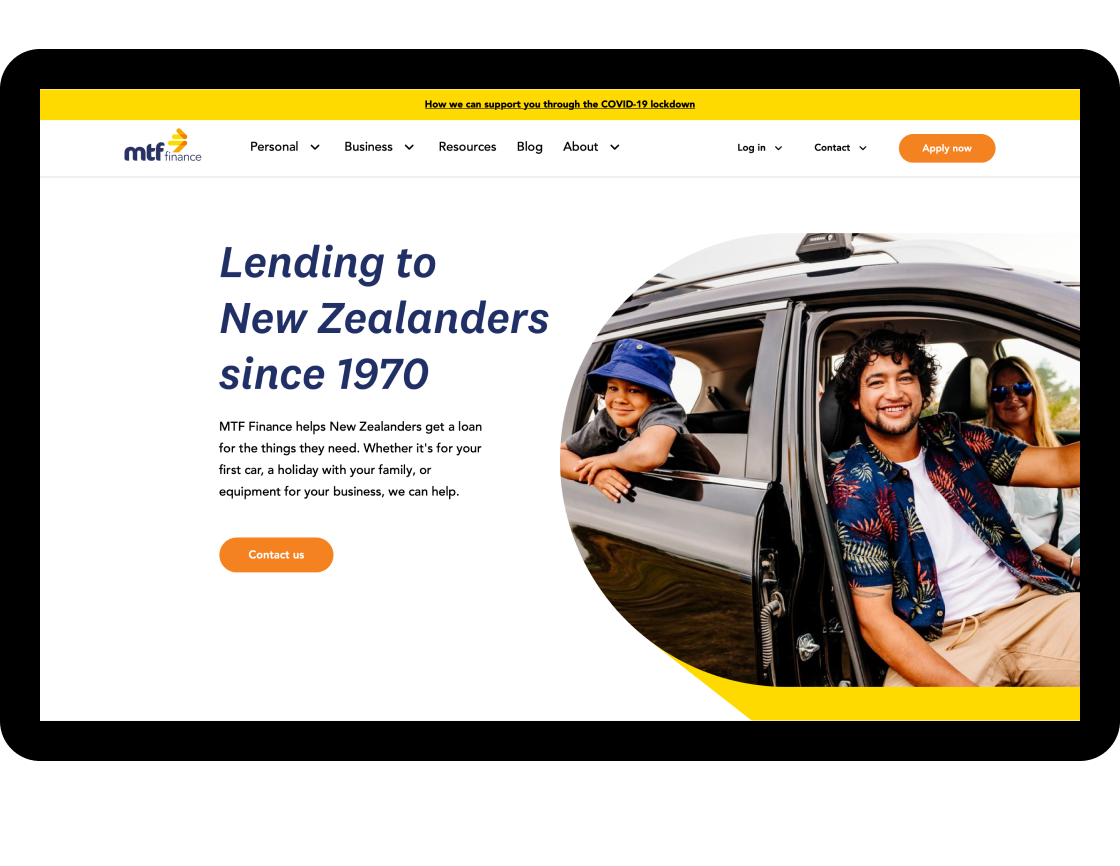A banner with a bright yellow top bar features black text that reads, "MTF Finance Personal, Business Resources, Blog, About, Login, Contact, Notify Now." Beneath this, the text states, "Lending to New Zealanders since 1970." The text further elaborates on how MTF Finance assists New Zealanders in obtaining loans for various needs, whether it's purchasing their first car, planning a family holiday, or acquiring business equipment. The call to action encourages viewers to contact MTF Finance for assistance.

In the accompanying image, a man with a vibrant Hawaiian shirt over a white t-shirt and tan pants is driving a vehicle. Beside him, a woman wearing a white shirt and sunglasses is seated with her seatbelt securely fastened. In the backseat, a little boy wearing a blue hat gazes curiously. Notably, the man and the boy are both without seatbelts. The scene embodies a casual, family-oriented atmosphere. For more information, the caption directs to visit www.mtffinance.co.nz.